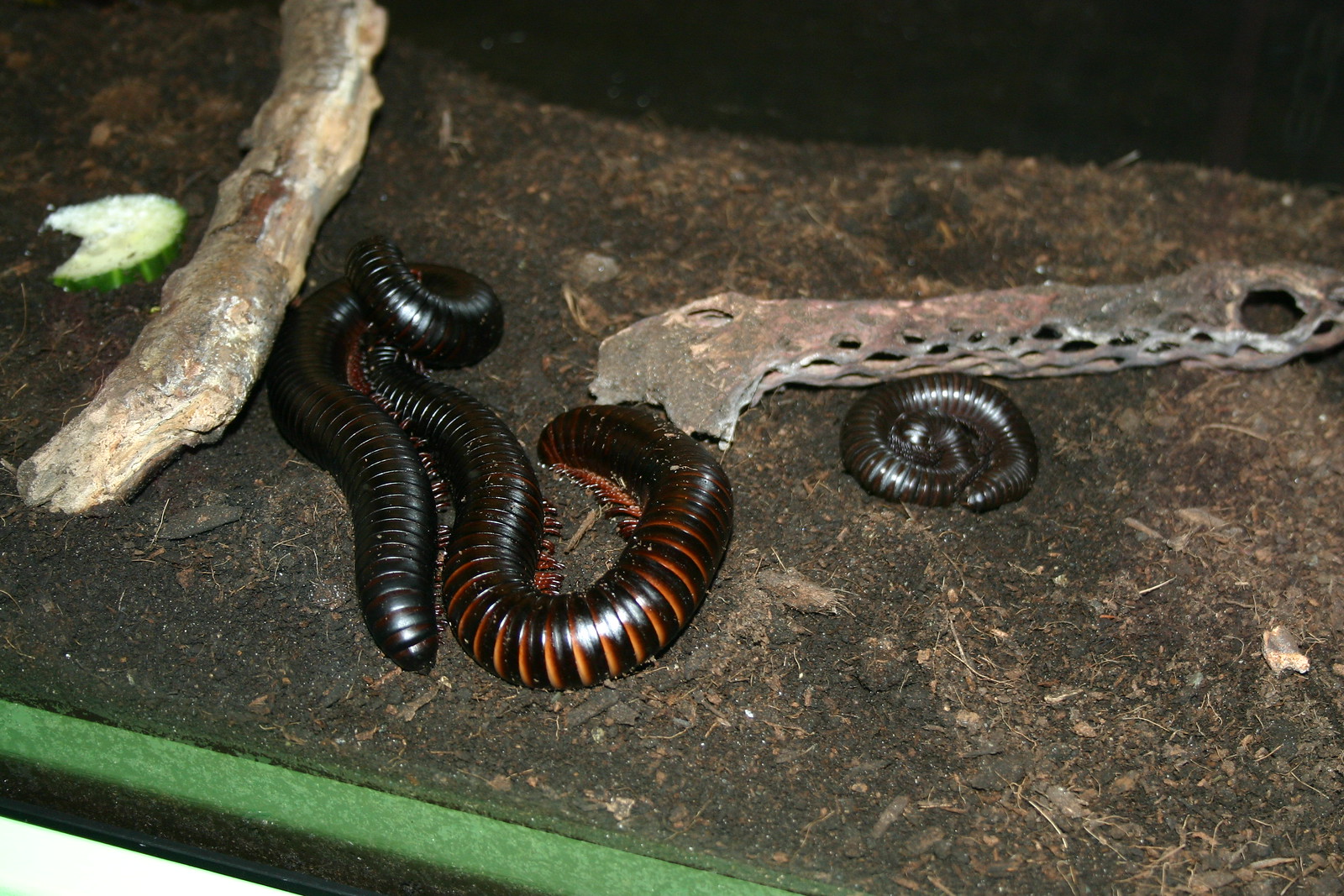The photograph captures a close-up scene inside a terrarium, which is set on a green felt surface. Visible through the transparent glass front, the terrarium’s interior is filled with dark brown soil scattered with various pieces of wood and vegetation, providing a naturalistic backdrop. Towards the left of the image, a cucumber slice with green edges and a white center lies partially eaten, adding a pop of color to the earthy setting.

Dominating the scene are three long, segmented millipedes—two larger ones with striking black and orange banded bodies adorned with numerous legs, and a smaller, similarly colored one, which is partially coiled. These millipedes are positioned next to a gray and white tree branch within the terrarium. The image, likely taken under artificial lighting, emphasizes the intricate details and textures of the millipedes and their environment, making it a fine example of nature photography.